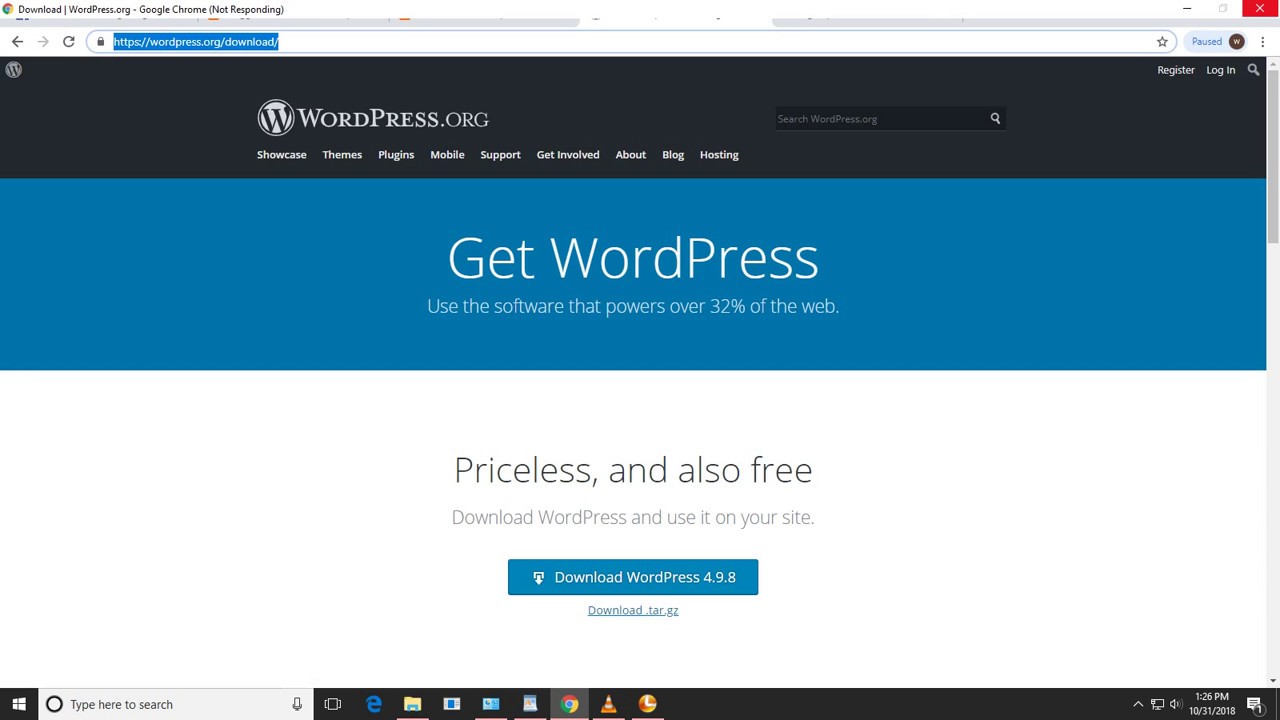The image depicts the WordPress.org Download page viewed on the Google Chrome browser. In the upper left corner, the browser tab shows "Download – wordpress.org" followed by a status indicating "Not Responding" in parentheses. The browser's interface includes a back arrow, a grayed-out forward arrow, and a Refresh button. The address bar is displayed with the URL "wordpress.org/download," confirming that the user is on the Download page of the WordPress website. The site features a black navigation bar stretching from left to right, containing the WordPress.org logo, the site title, and a horizontal menu. This menu includes options like a search bar, a Register button, a Login button, and a magnifying glass icon.